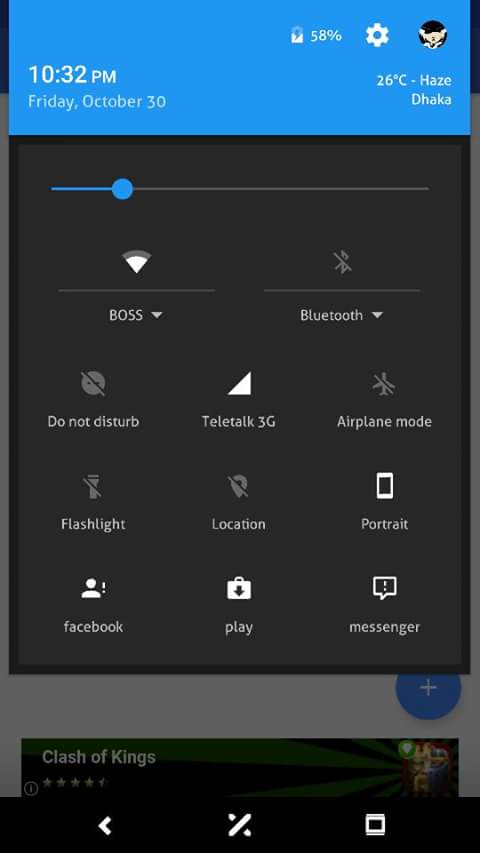This is a detailed screenshot of a smartphone's settings menu. At the top, it displays the current time, date, battery level, a profile picture, temperature, and location. The menu allows for various adjustments:

- **Brightness:** An adjustable spectrum slider enabling precise control over screen brightness.
- **Wi-Fi:** Shows the device connected to the "BOSS" Wi-Fi network.
- **Bluetooth:** A toggle to enable or disable Bluetooth connectivity.
- **Do Not Disturb Mode:** An option to mute notifications.
- **Network:** "Teletalk 3G" indicates available cellular connectivity options.
- **Airplane Mode:** A toggle to disable all wireless communication.
- **Flashlight:** An option to turn on the device's flashlight.
- **Location Tracking:** Toggle to enable or disable location services.
- **Portrait Mode:** An option for screen orientation settings.
- **Facebook, Play, Messenger:** Quick access icons for specific apps.